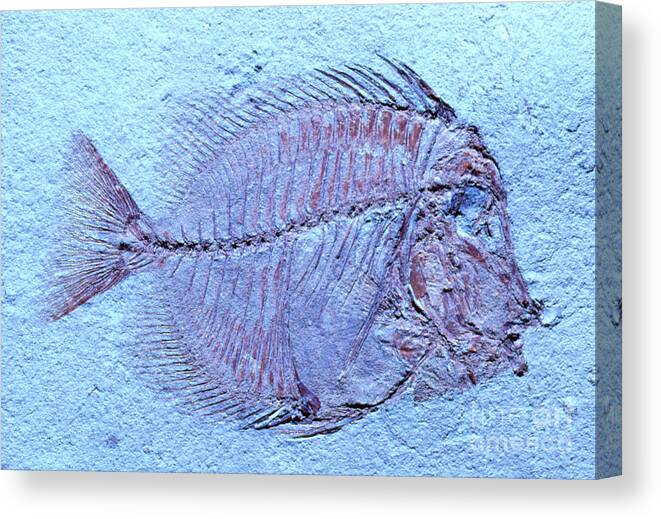The image depicts a high-quality product photograph intended for online commercial use, such as for shops, catalogs, or websites. Set against a solid white background and surface, the central focus is a rectangular-shaped canvas print showcasing a fossilized fish. The canvas edges are also printed, giving it a seamless, three-dimensional appearance as the print continues around the sides. The fish fossil, centered on a textured light blue rock-like background, reveals the skeleton and outline. The fossil features thin, spiny ridges along its back and stomach. The fossil itself displays a disc-shaped body with its face turned to the right and tail pointing left. This canvas wrap print adds a sculptural quality to the piece, enhancing its visual depth. In the lower right corner, a faint white signature is visible, and a Fine Art America watermark is present in the bottom left corner, indicating the marketplace from which this artwork is sold.